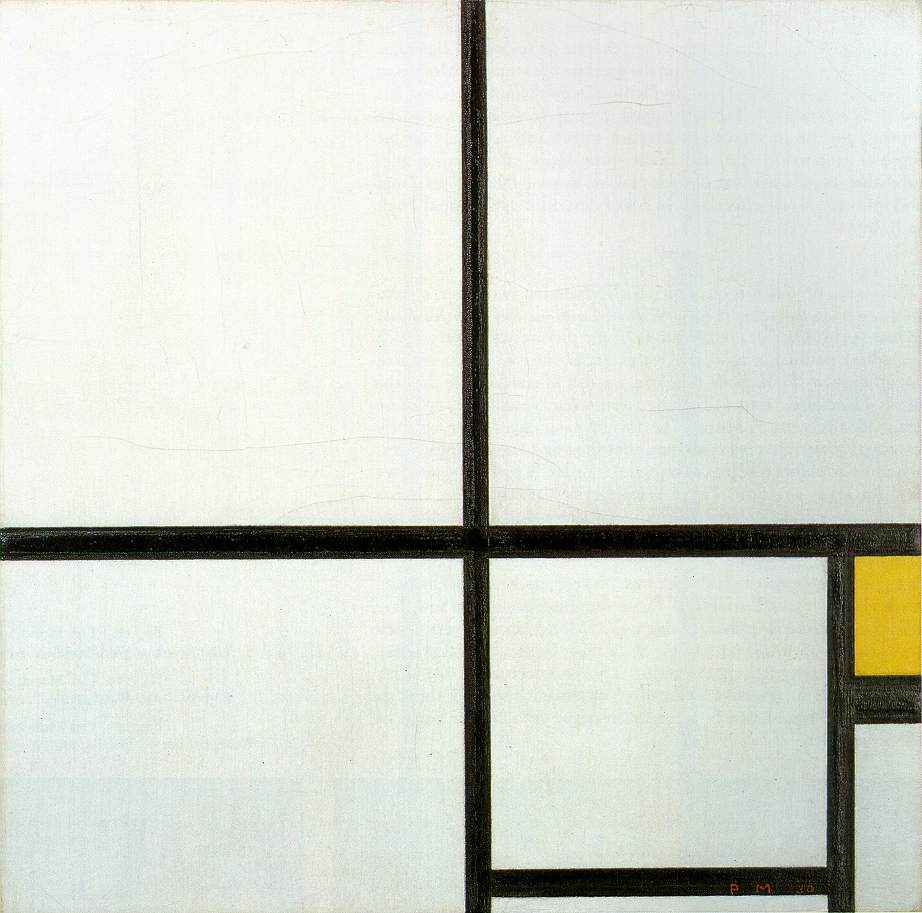This abstract, pattern-based artwork features a predominantly white backdrop intersected by various black lines, creating a geometric composition. The primary focus is a thick black vertical line that extends from the top to the bottom of the piece. Roughly a third of the way down, a slightly wider horizontal black line intersects the vertical line, forming a cross. This division of space results in four distinct quadrants. The bottom right quadrant is notably more intricate, featuring additional patterns: there is a smaller white square and adjacent to it, a smaller, bright mustard-yellow rectangle. Both shapes are framed by the black lines, which also display subtle variations in shade, including hues of gray and off-white. In the bottom right-hand corner, one can faintly discern what appears to be a scrawled signature or text, potentially reading "p.m. 56," though it is difficult to decipher clearly. The interplay of lines and colors, along with the subtle textual element, adds depth and intrigue to this enigmatic piece.